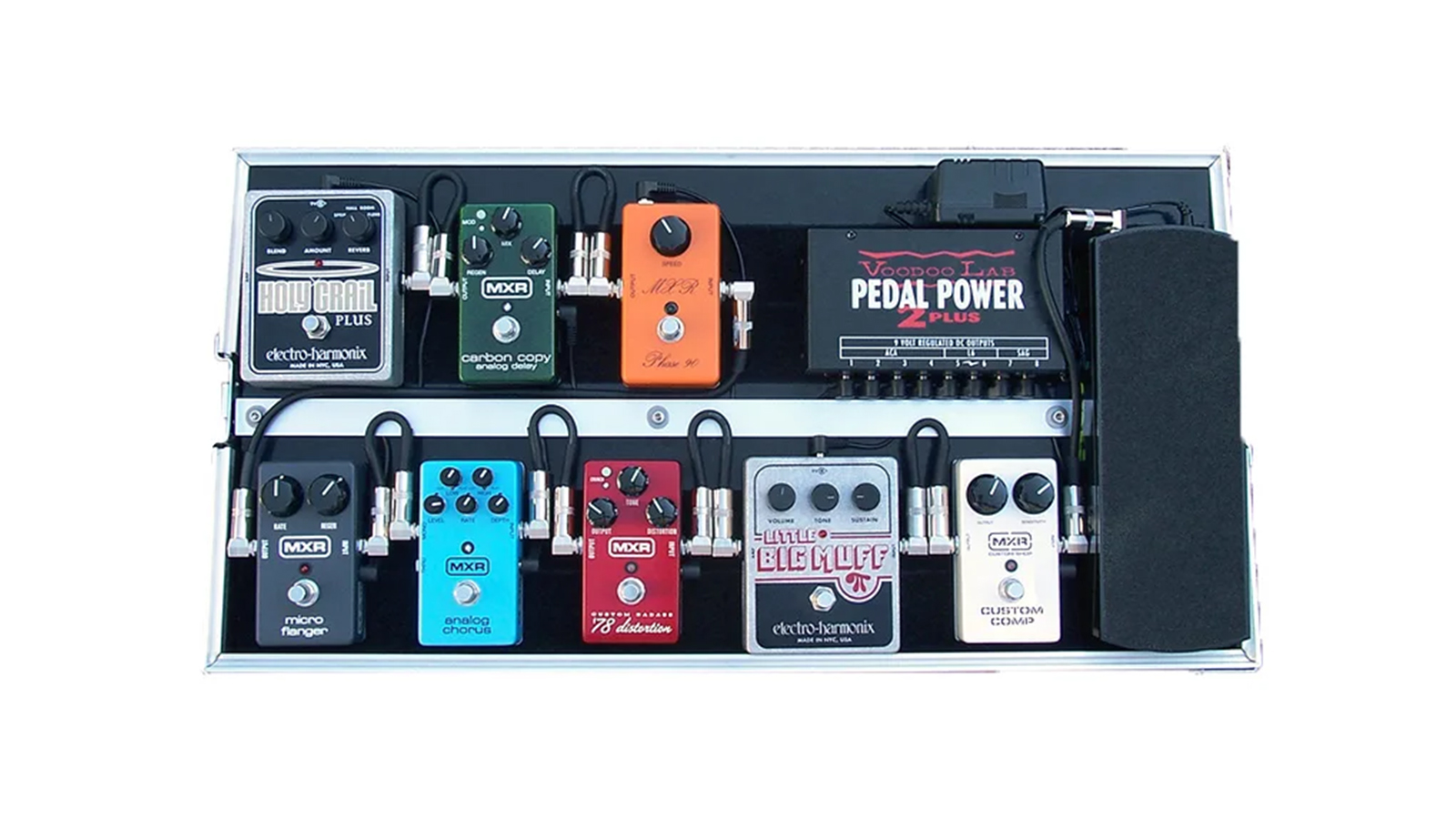A meticulously captured bird's eye view photograph showcasing the Voodoo Lab Pedal Power Z+, a professional-grade pedalboard power supply. Each element of the sleek, black unit is clearly visible, highlighting the printed text: "Voodoo Lab Pedal Power Z+" in bold white lettering. This essential device for musicians, particularly guitarists, is designed to power multiple pedals simultaneously, ensuring optimal performance and noise reduction. Surrounding the central power supply, an array of diverse effect pedals can be seen, each equipped with various dials and switches. These controls allow users to fine-tune and blend different sound effects, enhancing the musical experience by adding layers of tonal intricacy. The arrangement and details captured in this photograph underscore the precision and functionality of this must-have piece of musical equipment.